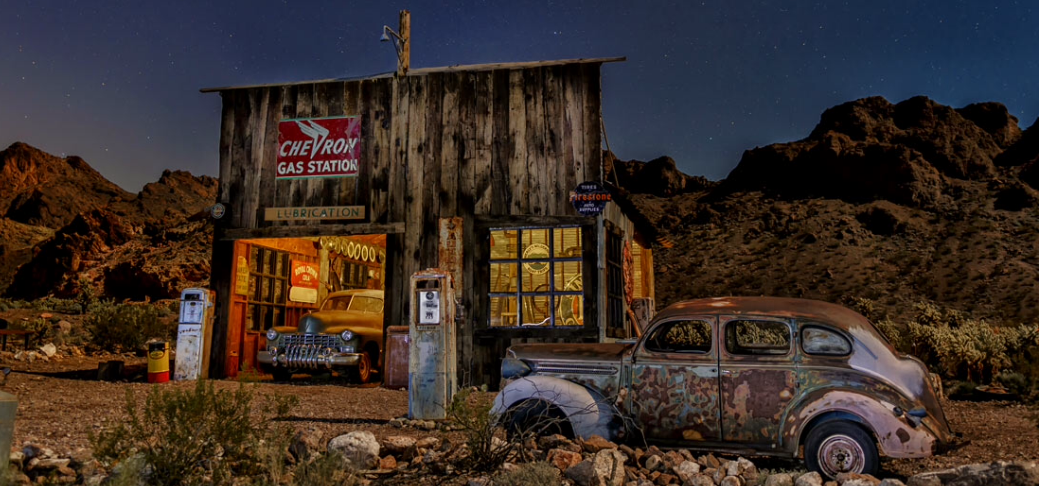The photograph captures a richly saturated, colorized image of an old and weathered Chevron gas station set against a desert landscape. The station, located slightly off-center to the left of the image, features a small wooden garage with an open door illuminated by a warm, inviting light. Inside the garage, the front end of an old vehicle is partially visible. Affixed to the top left corner of the building is a red sign with white lettering that reads "Chevron Gas Station," accompanied by a smaller sign below indicating "Lubrication."

To the right of the station, the building has nine-pane windows through which the interior glow can be seen. Scattered across the foreground are two gas pumps: one positioned about 10 feet in front of the Chevron station and another possibly an old air pump situated more to the left, near the garage. A heavily rusted, antiquated car with its windows missing—likely an elderly model Ford or Edsel—rests horizontally toward the lower right corner of the image, framed by some rocks.

The scene features a dirt road leading up to the station, with tall, craggy hills in the background beneath a vivid blue sky mixed with hints of dusk or a starry night, adding to the nostalgic and desolate atmosphere of the setting.